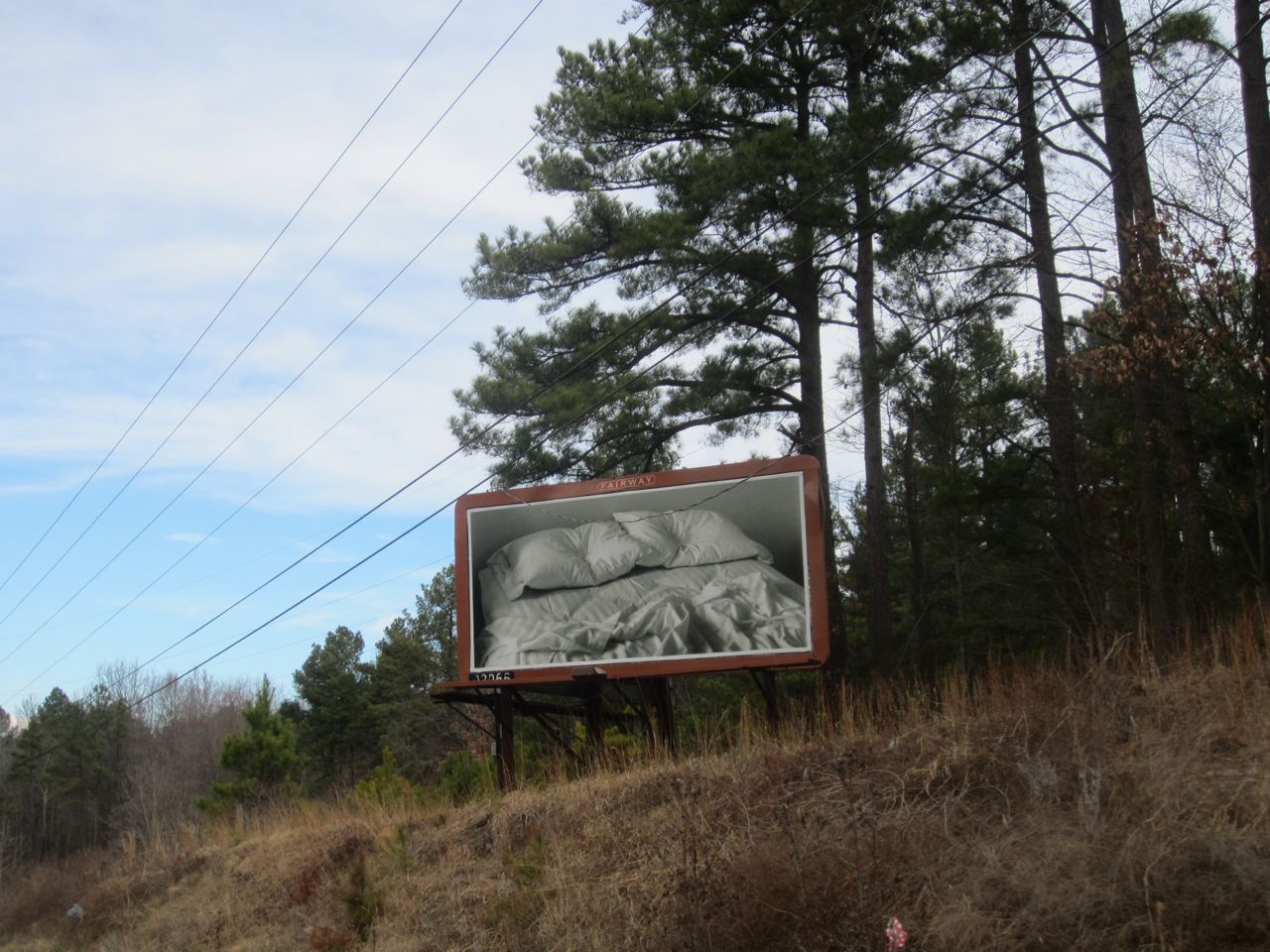The image captures a roadside billboard seen from a ground-up perspective. The billboard stands atop a steep, rugged, brownish slope covered in sparse, dying wild grass. Beyond the billboard, tall trees form a dense backdrop, while telephone wires angle diagonally from the bottom left to the top right of the frame, adding an element of structure to the scene. The sky above is a clear blue with some wisps of clouds, indicating a pleasant day. The billboard itself is bordered in red and prominently displays the word "Fairway" at the top. In the bottom left corner of the billboard, a small black box features the number "12066." The main visual on the billboard is a bed adorned with two somewhat flattened white pillows and a white bedspread atop a white mattress, all appearing wrinkled and well-used.